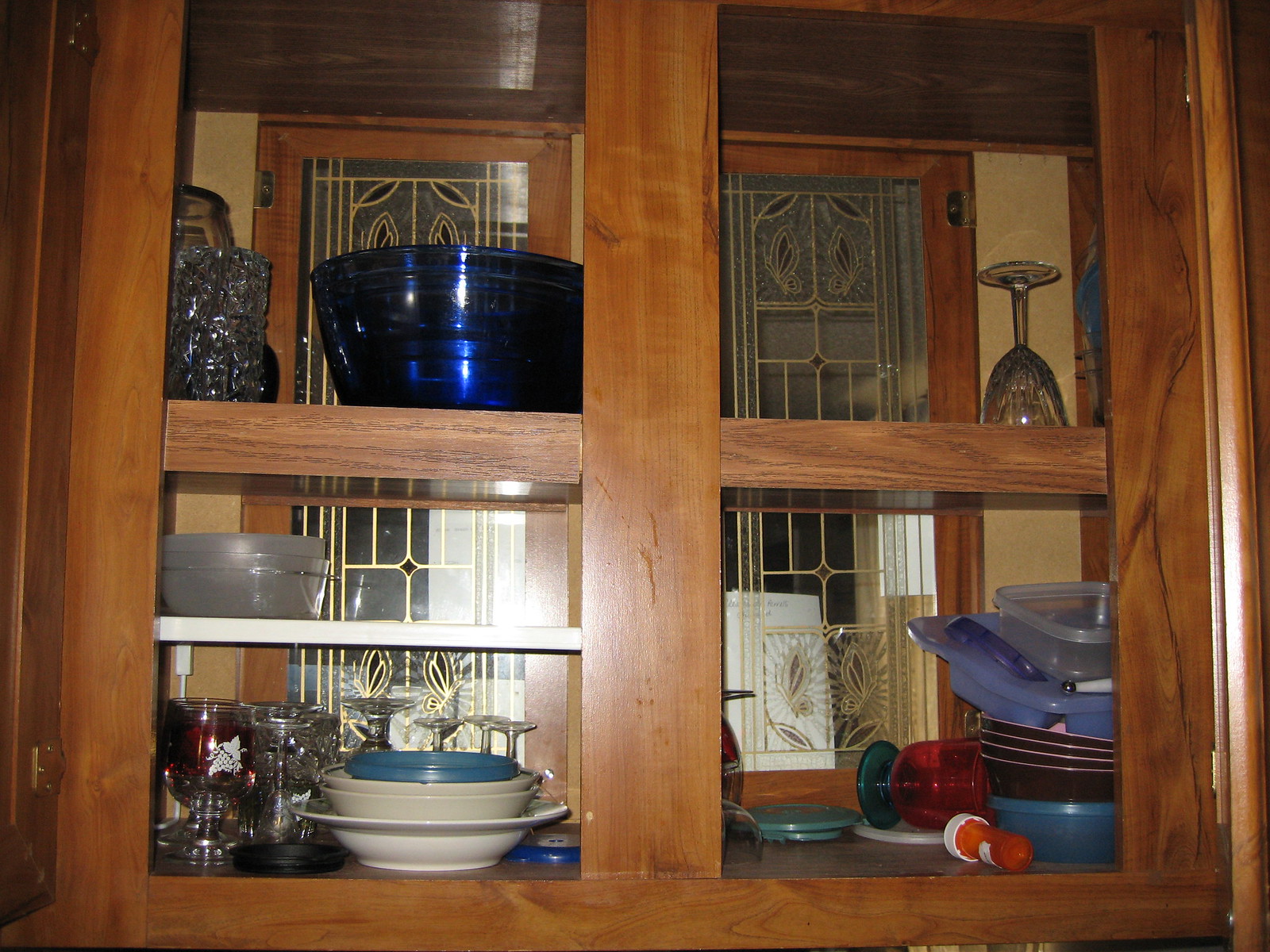A well-organized wooden cabinet with a bristly patterned glass back and multiple shelves. The top shelves contain an array of glassware, including a collection of neatly stacked blue glass bowls on the left, a set of inverted glasses on the far right, and a clear bowl with a white stripe in the center, illuminated by soft white light. The bottom shelves feature various plastic containers, starting with a stack of bowls at the bottom right, transitioning to square containers above them. Centrally placed is an orange pill bottle with a white cap. On the far left of the bottom shelf, there are white bowls filled with small blue balls, with additional glassware placed strategically around the cabinet. The intricate divisions and multiple lines of the glass pattern add a touch of elegance to the overall appearance of the cabinet.